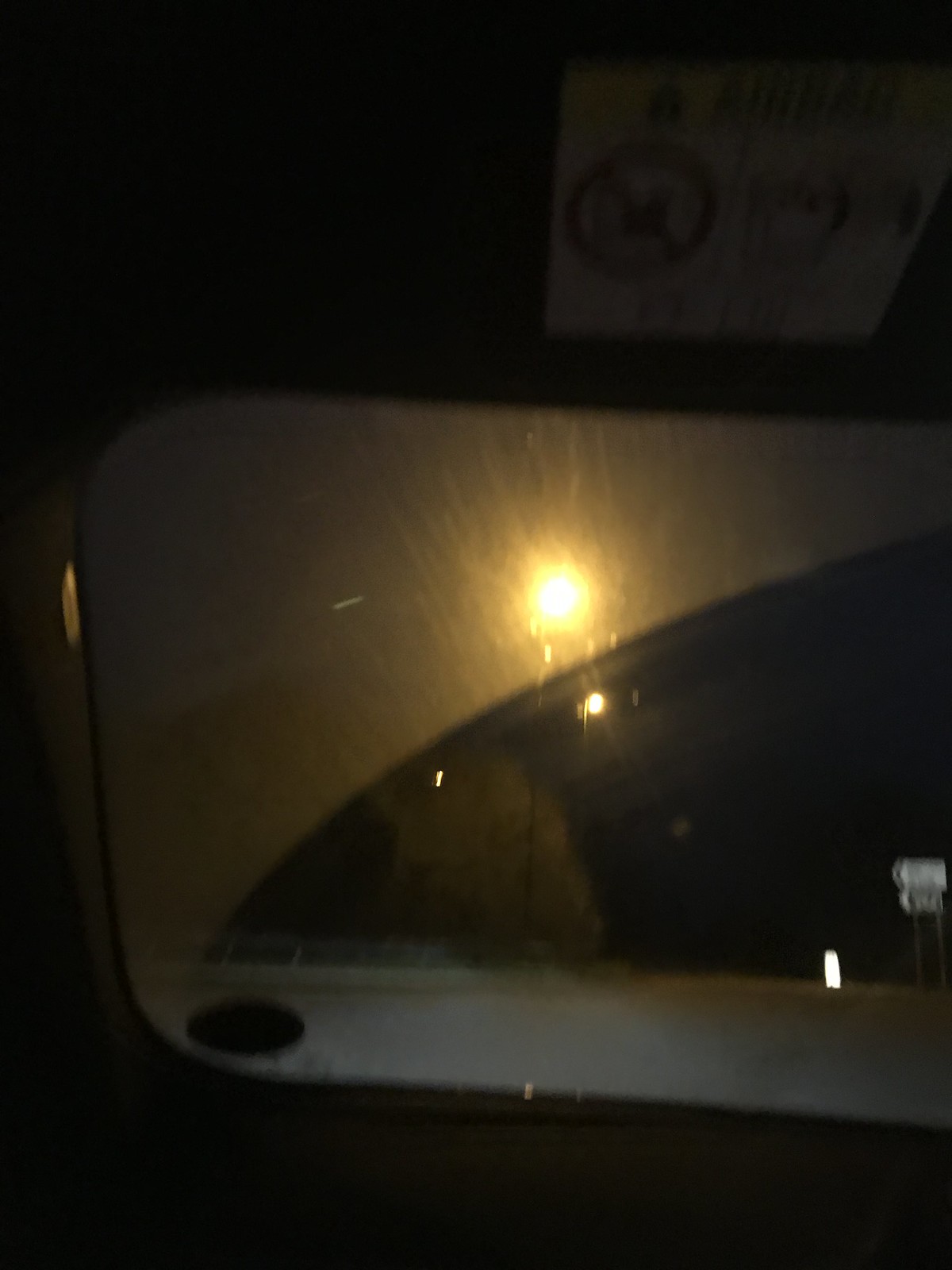This nighttime photograph captures a mysterious and moody scene, most likely taken from within a vehicle. The dominant feature is a rearview mirror, which reflects the bright headlights of a car trailing close behind. The artificial light from the headlights pierces through the surrounding darkness, casting an eerie glow that highlights the mirror's frame. This frame delineates the boundary between the illuminated area and the obscured edges, adding depth to the photograph. The interplay of shadows and light suggests a silent, nocturnal journey, followed closely by another vehicle.